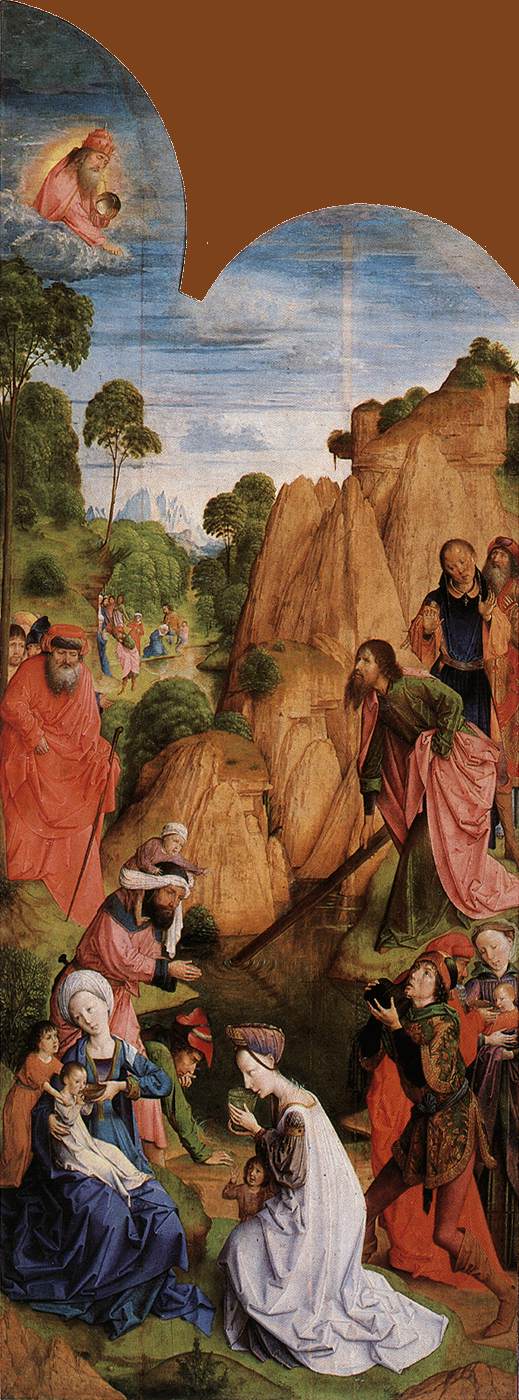The image is a vibrant, detailed painting, likely from the 15th or 16th century, with rich hues of oranges, browns, and yellows. Shaped as a tall rectangle, it exudes biblical and holy imagery. In the upper left, trees outline the outdoor scene. Central to the composition is a divine figure, possibly Jesus or God, pointing downward. Below, various figures in medieval robes engage in different activities: a woman in a long, flowing blue robe feeds a baby on her lap, with another child nearby. Adjacent to her, a woman in a white robe holds a bowl to her mouth. A man, hands clasped as if in prayer, carries another child on his shoulders. Nearby, an older man also appears to be praying, directing his gaze upwards toward the divine figure. An individual in a rose-colored robe and headgear, imbued with a halo-like glow, underscores the painting's sacred theme. Other figures are engaged in everyday tasks, such as getting water and moving rocks, contributing to the image's dynamic scene of medieval life intertwined with spiritual reverence.